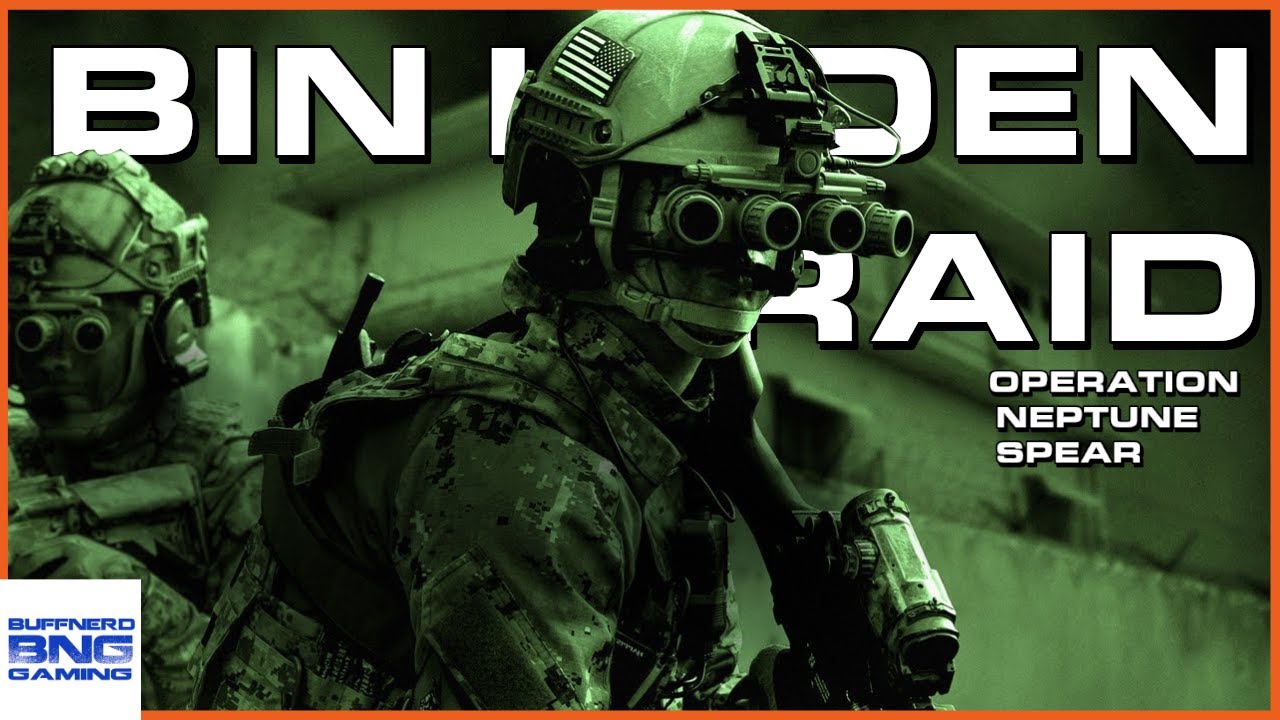The image appears to be an advertisement for a video game, framed horizontally with a thin orange border around its edges. The overall color scheme is predominantly green and black, reminiscent of night vision. The central focus is on two military soldiers depicted from the chest up, both clad in fatigues and helmets. The soldier in the forefront features an individual wearing an American flag on his helmet and equipped with what looks like a sophisticated binocular or eyepiece setup, featuring four circular lenses resembling those of a microscope. He also carries a weapon, which appears to be a laser gun, and dons a strap or bag across his body. Behind him stands another soldier, also equipped with a similar eyepiece. The background of the image hints at a building but remains obscure in the dark green tones.

Across the middle of the image, partially obscured by the soldiers, is bold white text reading "BEN LADEN RAID" with slight black shadowing, and underneath in a smaller font, it says "Operation Neptune Spear." In the bottom left corner, there is a white square containing a blue logo that reads "Buff Nerd BNG Gaming." The visual elements combined with the textual cues strongly suggest this is promotional material for a video game, focusing on a military operation.